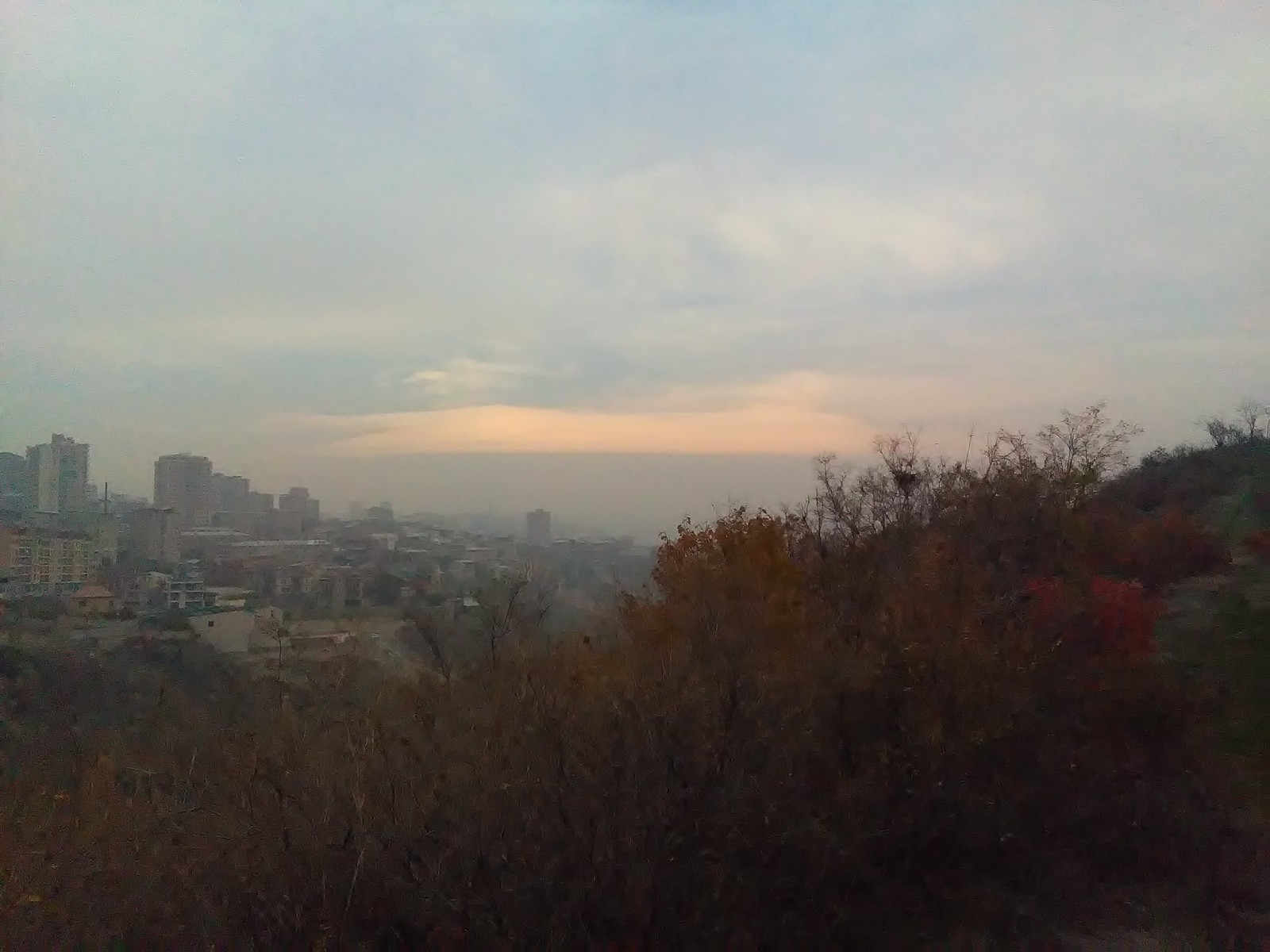The image captures an outdoor scene from a hilltop vantage point, overlooking a distant city. The foreground is dominated by dried-up brush and plants in hues of orange, brown, and dark red. The sky above is a dimly lit blue, interspersed with gray, overcast clouds, adding a certain gloominess to the lighting. The left side of the image prominently features the city skyline with several large, yet not towering, skyscrapers partially obscured by a light haze, hinting at possible rain. The right side is dominated by the hilltop itself, devoid of any pathways, making it appear as a random, natural hillside. In the far distance, another hill mirrors the one in the foreground, while industrial areas stretch between the two hills, adding an urban contrast to the natural elements.